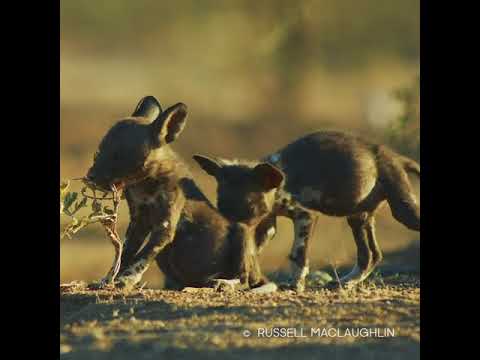This nature photograph, attributed to Russell McLaughlin in white font in the bottom right corner, captures two small, possibly canine animals with pointy ears reminiscent of foxes. They have a distinct coloration with dark brown fur, accented by white spots on their front paws. Against a backdrop of dry, earthy terrain and a hazy gradient of greenish-brown, the scene is framed on the left and right by black vertical borders. The animal on the left, appearing to chew on a dying small tree or sapling with green leaves and a brown trunk, exhibits a curious demeanor, while the animal on the right seems to be sniffing the other’s backside.